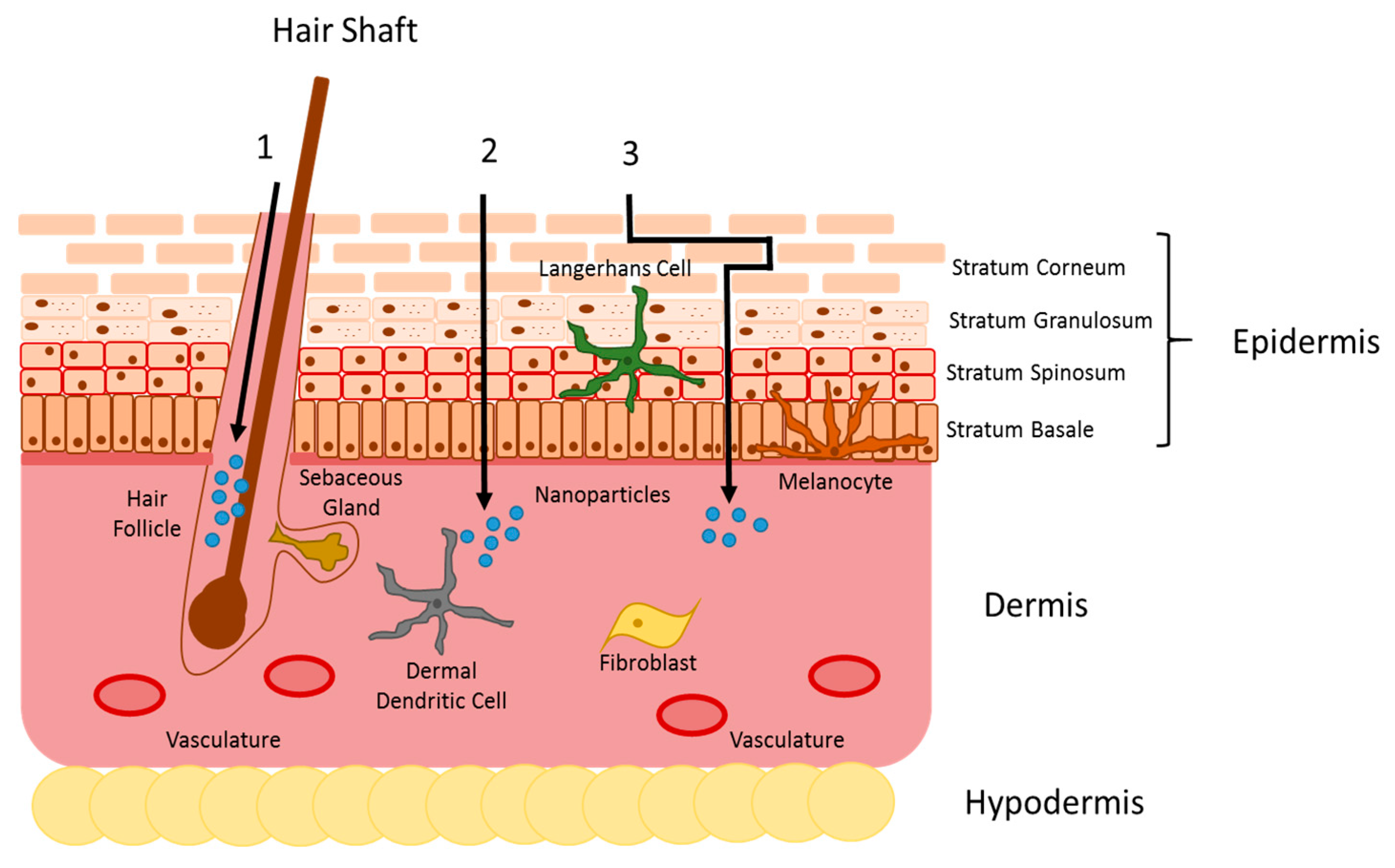This detailed illustration depicts a hair shaft and the surrounding structures as they exist below the skin's surface. The diagram, set against a white background, uses vibrant colors such as pink for the dermis, green for highlights, and beige or yellowish for the hypodermis layer. The image features a labeled cross-section of the skin, with the hair shaft extending down into the hair follicle and sebaceous gland located nearby. The illustration highlights various cellular components and structures, including the dermal dendritic cell, fibroblasts, vasculature, melanocytes, and nanoparticles, specifically labeled at points numbered one, two, and three. The epidermis and the subsequent layers of the skin—dermis and hypodermis—are clearly labeled to the right of the image. The chart is laid out in a textbook-style format, with colorful depictions and precise labels such as the Langhorn cell shown in green, making it a comprehensive visual representation of the hair follicle and its surrounding tissues.